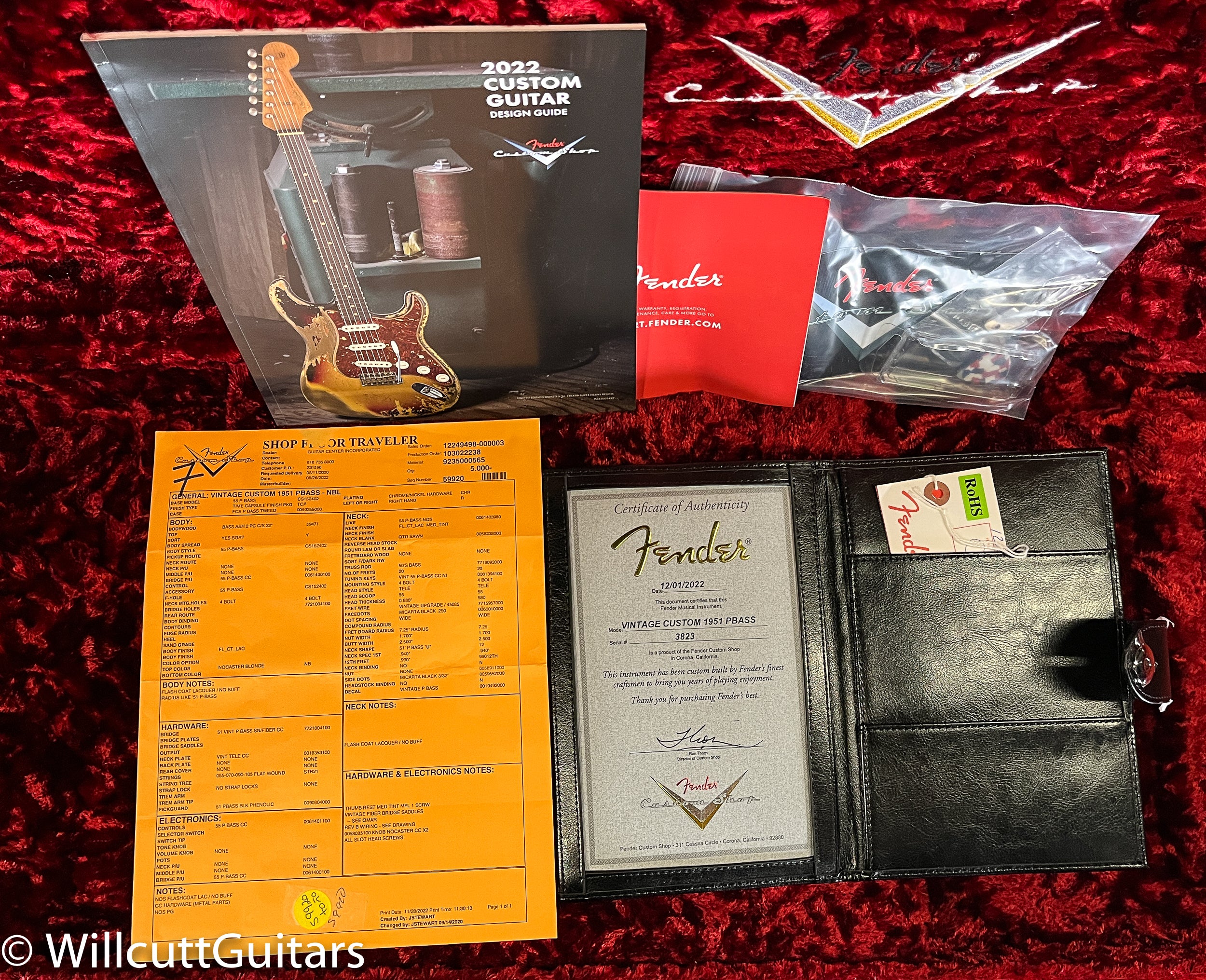This is an overhead, flat lay marketing photograph highlighting a collection of materials accompanying a brand new Fender guitar, all set against a rich, deep maroon crushed velvet background. 

In the upper left corner, there's a 2022 Custom Guitar brochure featuring a photograph of a Fender Stratocaster on the cover, adjacent to white text and the Fender logo, which consists of a chevron V with "Fender" in orange and "Custom Guitar" in handwritten script in white.

Moving to the right, a clear cellophane package with a red label is visible, containing various accessories like guitar strings, picks, and possibly fret wires. This package bears the detailed Fender branding, featuring the iconic script lettering.

On the right side of the arrangement is a black leather portfolio opened flat. The left side of the portfolio displays an official Fender Certificate of Authenticity, complete with the Fender script logo, detailed information about the guitar, and a serial number. The right side features a pocket holding a Fender business card.

Below this setup, there is a bright orange order sheet, densely packed with rows of black text that details customization options and accessories for the guitar. This sheet prominently displays the Fender logo in the upper left corner.

Finally, nestled in the very bottom left corner, the image includes the copyright credit for "Willcutt Guitars," underscoring the authenticity and attention to detail of this custom Fender presentation.